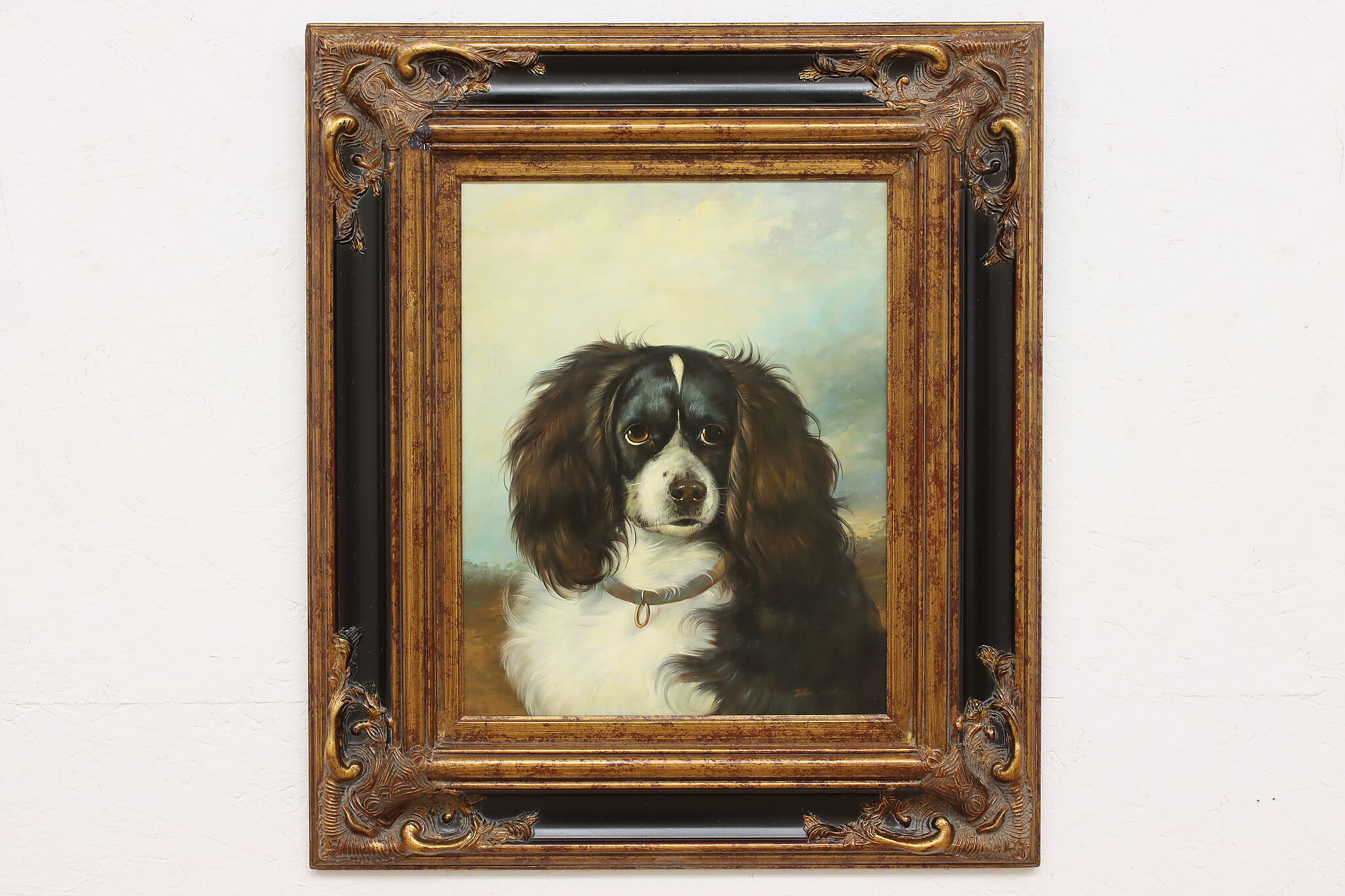The image depicts an ornate wooden frame with intricate carvings at each corner and a black border framing a detailed painting. Inside the frame, against a backdrop of a light blue sky with white clouds and brown fields resembling wheat, there is a portrait of a Cocker Spaniel dog. The dog, wearing a brown leather collar, is gazing slightly to the left with a somewhat blank expression. It has long, floofy ears with a brownish copper tint, a black and brown coat, a white chest and snout, and a distinctive black nose and eyes. The craftsmanship suggests this is a custom portrait, capturing the typical features and character of a beloved Cocker Spaniel.